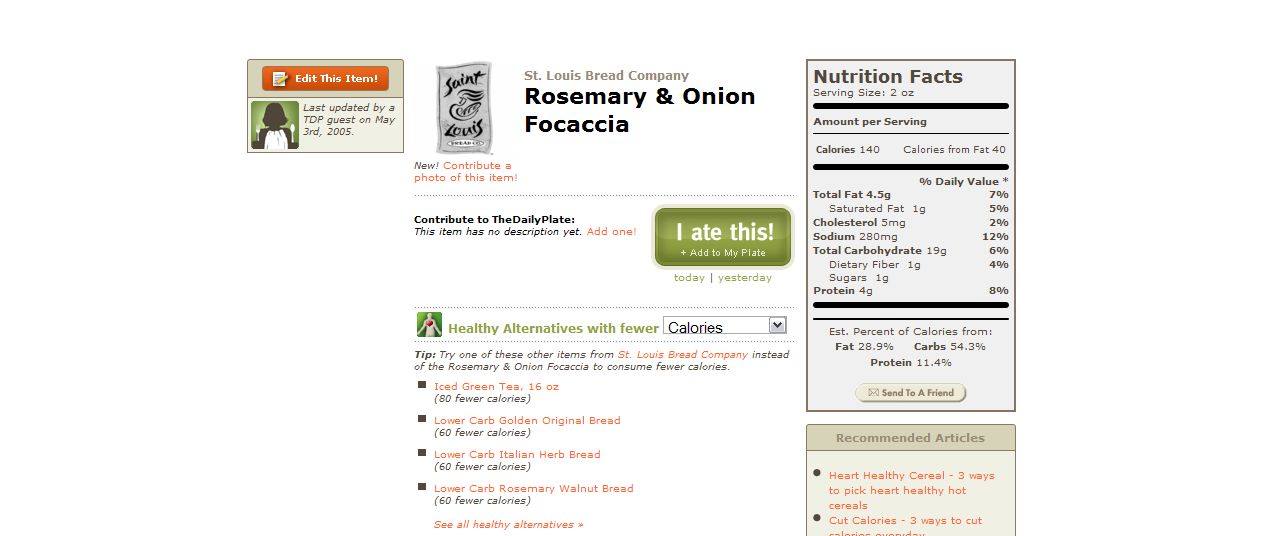This image is a detailed screenshot from a food or dieting website, likely The Daily Plate, providing information on St. Louis Bread Company's rosemary and onion focaccia. At the top, the page features a header "St. Louis Bread Company rosemary and onion focaccia," accompanied by an emblem of the brand. Underneath, there's a clickable box labeled "edit this item," followed by text noting, "last updated by a TDP guest on May 3rd, 2005."

To the right side of the image, there's a large rectangle containing comprehensive nutritional facts in black font, segmented by thick lines into distinct sections. Details include serving size (2 ounces), calories (140), calories from fat (40), and percentages for daily values of total fat, saturated fat, cholesterol, sodium, total carbohydrate, dietary fiber, sugars, and protein. It also outlines the percentage of calories derived from fat (28.9%), carbohydrates (54.3%), and protein (11.4%).

The left side of the image likely features interactive elements such as a green box with white text reading "I ate this. Add to my plate," indicating user engagement for tracking food consumption. Beneath this are reviews, visible in red font, and a silhouette image of a person with a fork and knife set against a green background.

Further down, a section titled "healthy alternatives" offers lower-calorie substitutes from the same restaurant, such as iced green tea (80 fewer calories), lower-carb golden original bread (60 fewer calories), lower-carb Italian herb bread (60 fewer calories), and lower-carb rosemary walnut bread (60 fewer calories). There's also an option to view all healthy alternatives.

The page provides additional tools like a box to send the information to a friend via email, links to recommended articles about heart-healthy cereal and calorie-cutting tips, and an interactive prompt to contribute a photo of the item or add a description, emphasizing user participation.